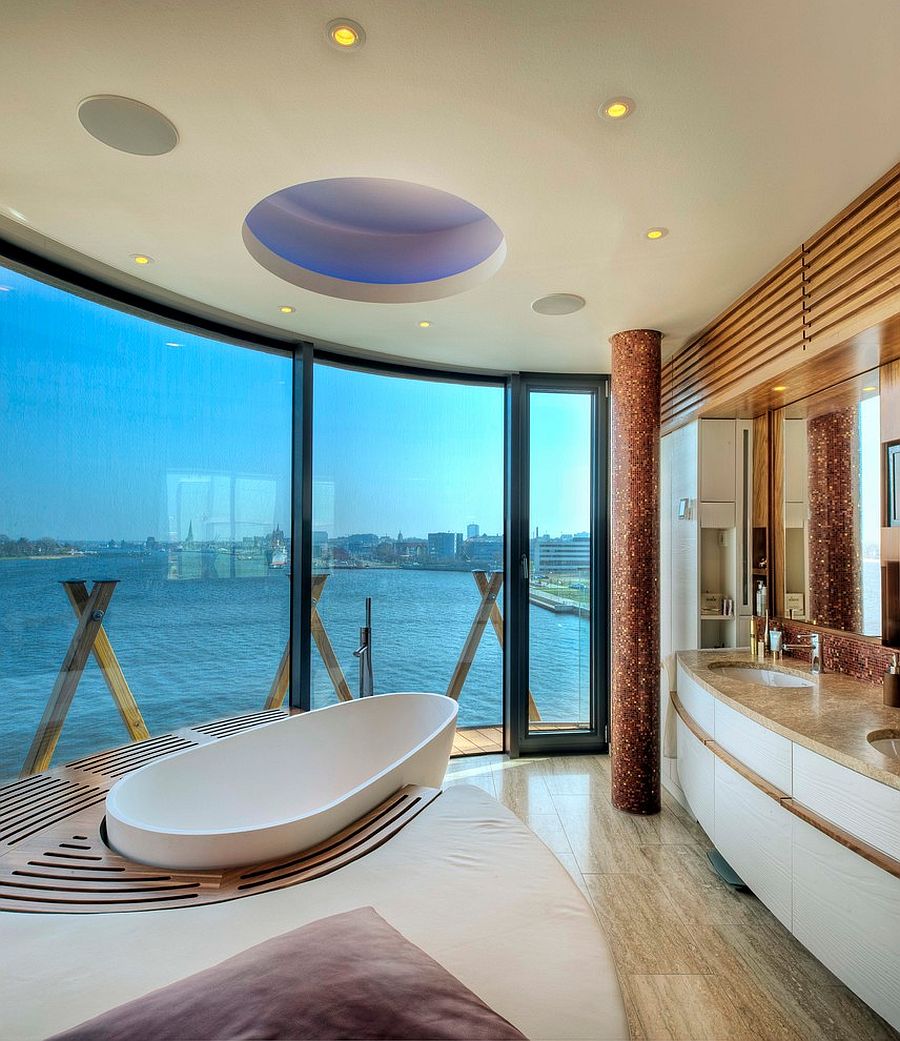This photograph depicts a luxurious, modern bathroom with a breathtaking waterfront view, possibly from a penthouse hotel suite or a high-end seaside residence. The room features floor-to-ceiling, curved, bluish-tinted glass windows that offer an uninterrupted vista of a clear blue sky, a large body of water, and a distant city skyline. A visually striking, oval-shaped, egg-like white bathtub occupies the center of an elevated platform made from teak or bamboo, surrounded by a white rug with a gray triangle design.

To the right, sleek cabinetry with strong lines supports a double sink with a granite top, framed by a large mirror and additional cabinetry. The ceiling is embellished with a skylight and circular recessed lighting. Dominating the room are tall, round, sparkly copper-colored pillars, adding a touch of glamour. The floor is covered in travertine, and there's a wooden seating area around the bathtub.

Notably, the design curves gracefully to follow the room’s overall circular motif, including the curved glass wall. The vanity and cabinetry mirror this curvature, enhancing the room’s cohesive elegance. The bathroom’s light brown and white color palette completes its sophisticated appearance.